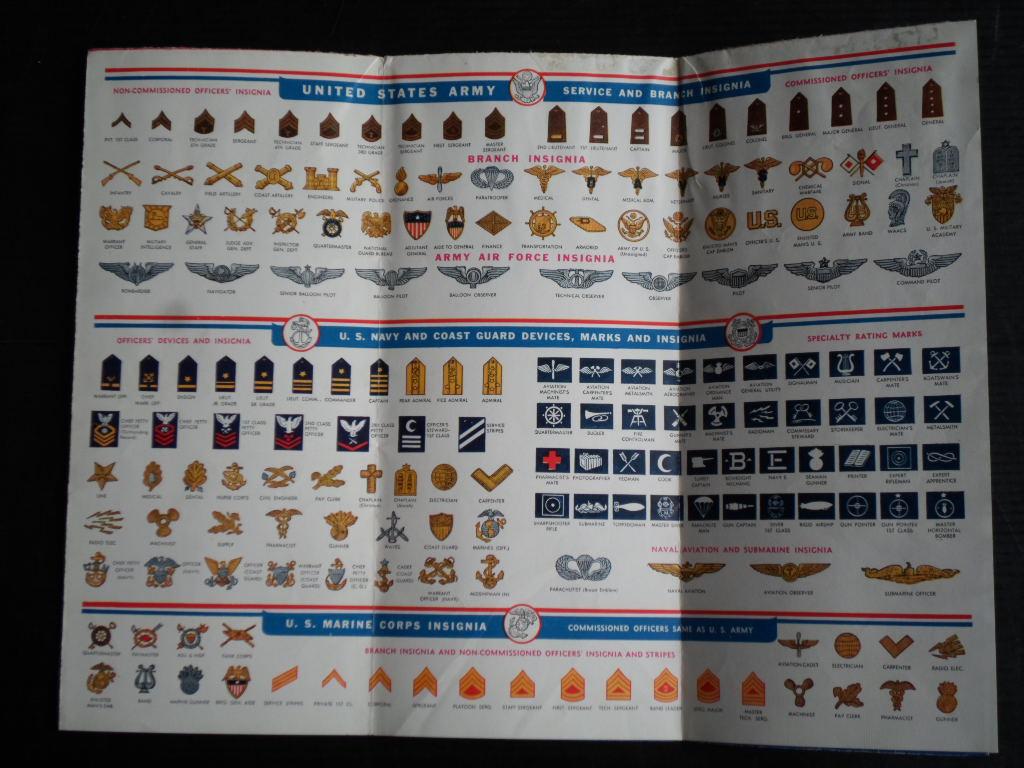This horizontal rectangular image features an open, folded pamphlet with a white background, densely packed with information relevant to military symbols, rankings, and insignia. At the top, the text reads "United States Army," "Service," and "Ranking," although some smaller print is hard to read clearly. The pamphlet is divided into three sections, each detailing different aspects of military identification and decorum. The middle part includes a collection of various signal flags used for communication. To the side, there are displays of medals and decorations, organized neatly in rows, with smaller badges on the far left gradually increasing in size towards the right. The bottom section demonstrates hand signals and features illustrations of faces adorned with different service hats. Additionally, there are patches and insignia specific to the U.S. Navy and Coast Guard devices, as well as Marine Corps insignia, all set against a vibrant palette featuring shades of orange and yellow. The level of detail and colorful presentation suggests this is an educational or reference material for understanding military insignia and decorations.